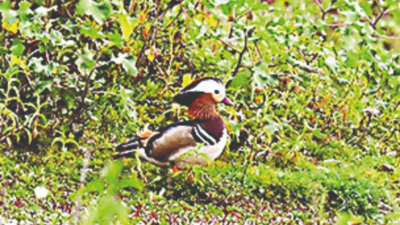In this picture, we see a small bird standing in the middle of a grassy field. The bird features a mix of colors: its top head is black, it has a bright red breast and beak, and white parts on its belly and head. Additionally, there are distinct white stripes on its wings. The bird is facing its right side towards the viewer, standing still amidst a field that has green grasses with some patches of red. In the background, there is bushy shrubbery with leaves and branches in various shades, including green, yellow, and hints of orange, suggesting a sunny and vibrant day. The bright sunlight illuminates the scene, highlighting the vivid colors and casting a natural shine on the bird and its surroundings.